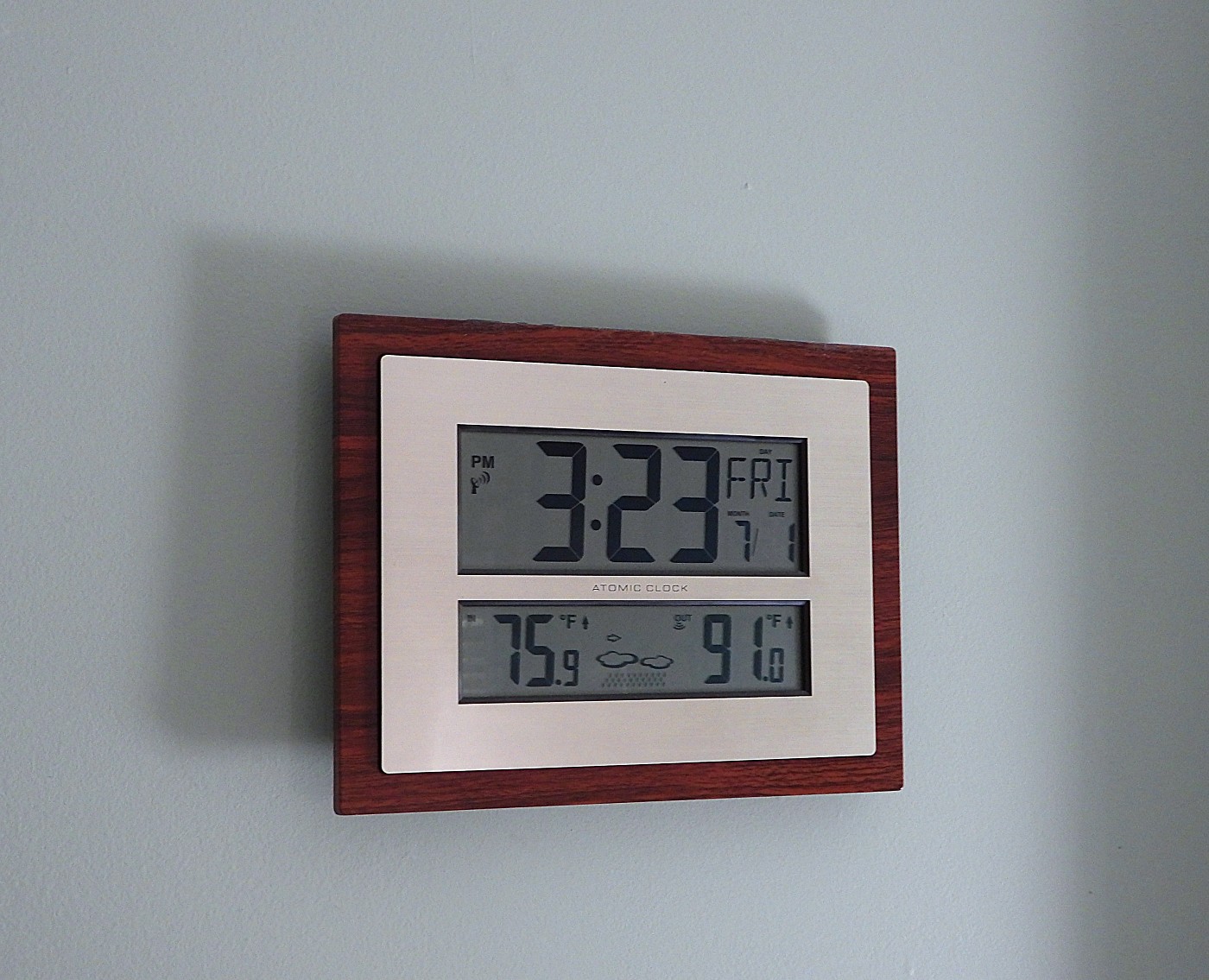The image showcases a rectangular atomic clock encased in a polished wooden frame, complemented by white framing surrounding two distinct digital display windows. The top window presents the precise time, showing 3:23 p.m. on a Friday, along with the date, which reads July 1st. The bottom window provides detailed environmental information, displaying an indoor temperature of 75.9°F accompanied by an upward-pointing arrow, and a weather icon featuring clouds and zigzag lines, possibly indicating rain. Additionally, the external temperature is noted as 91.0°F with another upward-pointing arrow. The clock, which functions as a multi-purpose device combining timekeeping, temperature measurement, and basic weather prediction, is elegantly mounted on a white wall adorned with an ecru paint in eggshell finish.